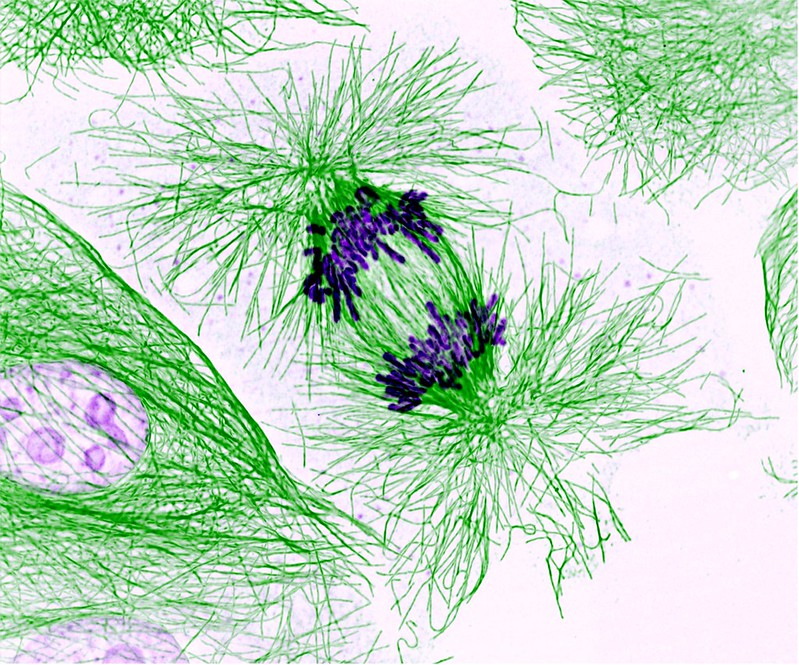This detailed illustration resembles a magnified pen drawing which captures the essence of a biological process intertwined with natural elements. The background is predominantly white, providing contrast against the intricate green lines that dominate the image. These green lines, resembling spindly grass or fine filaments, are scattered throughout the picture with clusters on the top right, top left, and middle sections. In the central area, there are two prominent structures composed of densely packed green filaments mixed with small, purple, flower-like elements. One of these central formations features a light purple circle embedded with smaller, darker purple circles, resembling a vacuole with intracellular components. Another notable feature towards the bottom left is a half-purple circle. The overall composition suggests a fusion between organic plant-like forms and cellular structures, with the green filaments extending outwards like grassy pom-poms or the twisted ends of a piece of hard candy, complete with ruffled edges. This blend of biological and botanical imagery gives the impression of looking through a microscope at a complex, dynamic process, potentially hinting at cell division or a similar phenomenon.